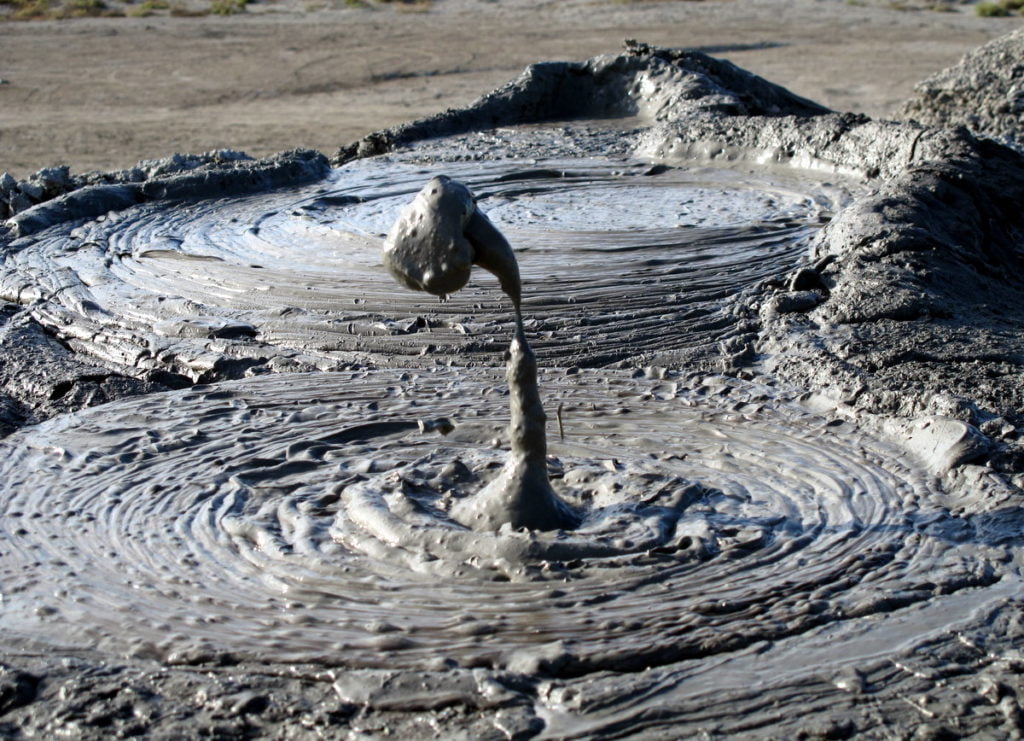The photograph captures a dynamic and intriguing muddy landscape. At its center lies an elevated pit of dark gray earthen sides, forming a stark boundary around two churning, bubbling pools of thick, viscous brown mud. The front pool is particularly captivating, with a large bubble of mud caught mid-air as it falls, reflecting the action and energy within the pit. The surface is marked with concentric rings and ripples, giving the impression of molten material. The rear pool appears more liquid, creating contrast with the thicker front pool. Surrounding the pit, a flat, barren brown plain stretches out indefinitely, under clear daylight. The composition suggests a sense of both movement and desolation, creating a raw and rugged natural scene.